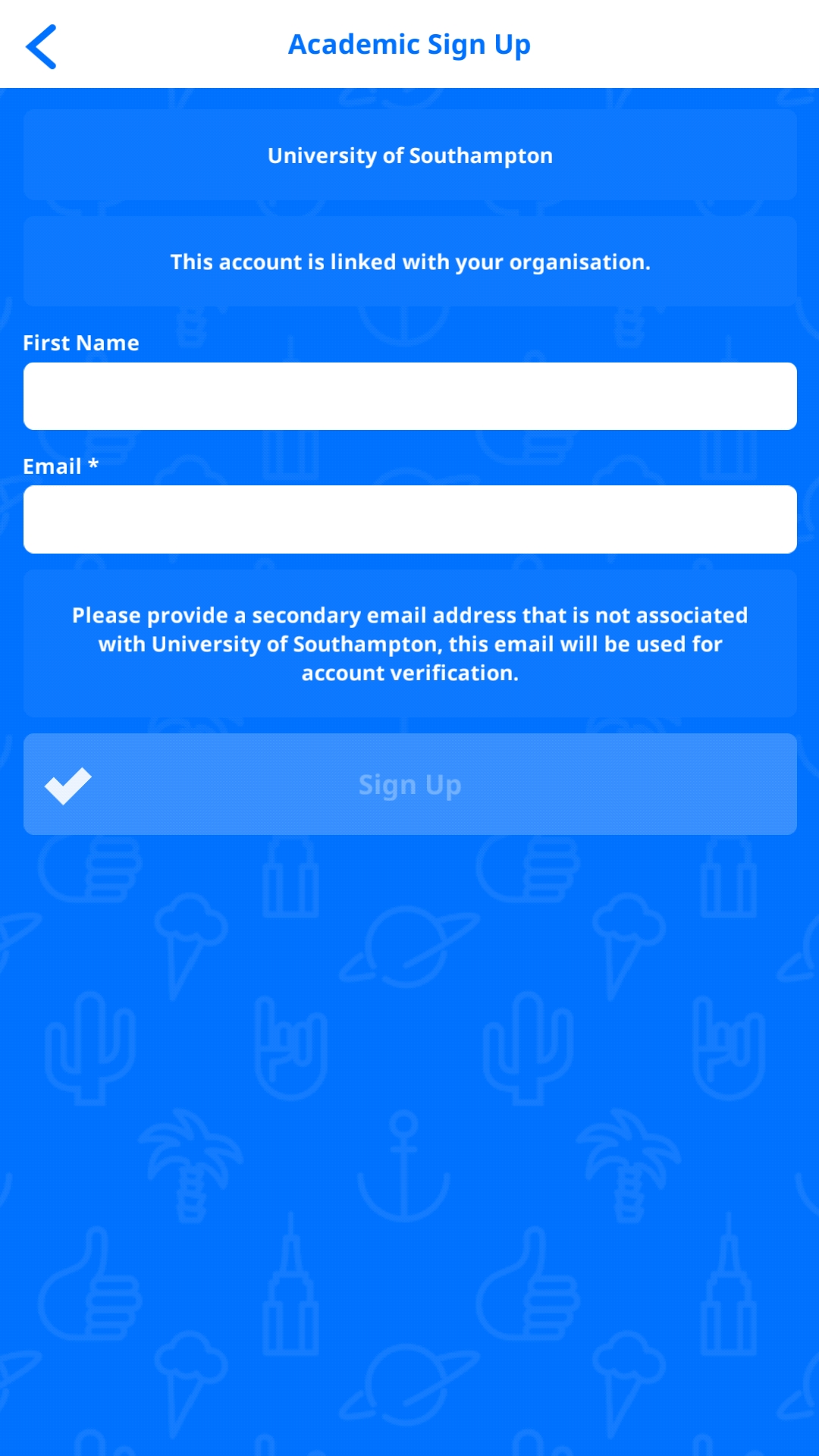The screenshot depicts the login page for the University of Southampton's academic sign-up portal. The interface features a predominantly blue and white color scheme. At the top of the page, there is a white header with a blue arrow pointing to the right, and the text "Academic Sign Up" appears in blue.

Below the header, the remaining menu area is filled with a blue background and white text. Prominently displayed at the top is the "University of Southampton" title, followed by a statement indicating that the account is linked with your organization. 

The login form includes two vertical white input boxes. The first box, labeled "First Name" in white text, is intended for the user's first name. The second box is labeled "Email" and has an asterisk indicating it is a required field. Beneath these fields, there is additional instructional text in white font on a blue background: "Please provide your secondary email address that is not associated with the University of Southampton. This email will be used for account verification."

At the bottom of the form, the "Sign Up" button is displayed in a slightly different blue rectangle, with greyed-out text and a white checkmark in the left corner, suggesting that the button is currently unclickable until all required fields are completed.

The background features a simple, symmetrical pattern in a very light blue shade, incorporating various icons such as an anchor, cactus, Saturn, thumbs-up, ice cream, and palm tree. The design is unobtrusive, ensuring that the text remains easy to read.